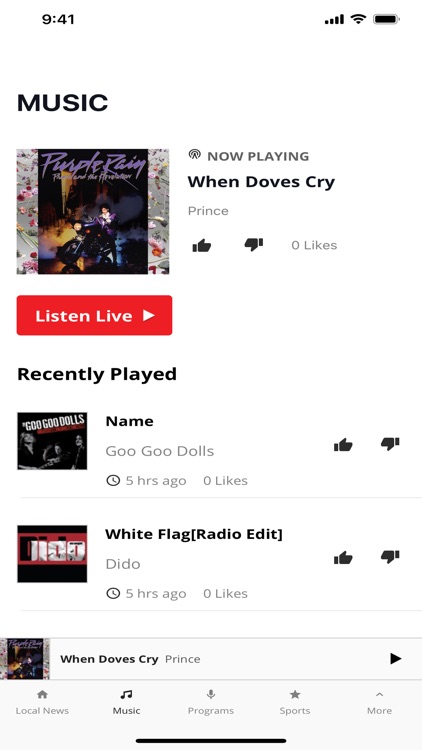The cell phone screen displays a music app interface against a white background. At the top, the header "MUSIC" is displayed in bold capital letters. The current time, 9:41, is shown in the upper left corner, and a fully charged battery icon is positioned in the upper right corner, both of which are bolded in black.

Below the header is the album cover of Prince's "Purple Rain", prominently featured, with the words "Now Playing" next to it. The song title, "When Doves Cry", is prominently bolded in black letters beneath the album cover, with the artist name "Prince" right below it in light gray letters. Thumbs up and thumbs down icons are displayed, indicating the song has zero likes.

Directly below the album cover is a short rectangular red banner with "Listen Live" written in white letters, accompanied by a white arrow pointing to the right. In bolded black below this banner is the label "Recently Played".

Two more album entries follow, each with the name of the album, the artist, how long ago it was played, the number of likes, and thumbs up/thumbs down icons. At the very bottom of the screen is a light gray banner displaying what is likely the currently playing song, "When Doves Cry" by Prince, along with the "Purple Rain" album cover once again. A bolded black arrow points to the right, inviting interaction. Additional text below this banner lists categories such as "Local News", "Music Programs", "Sports", and more.